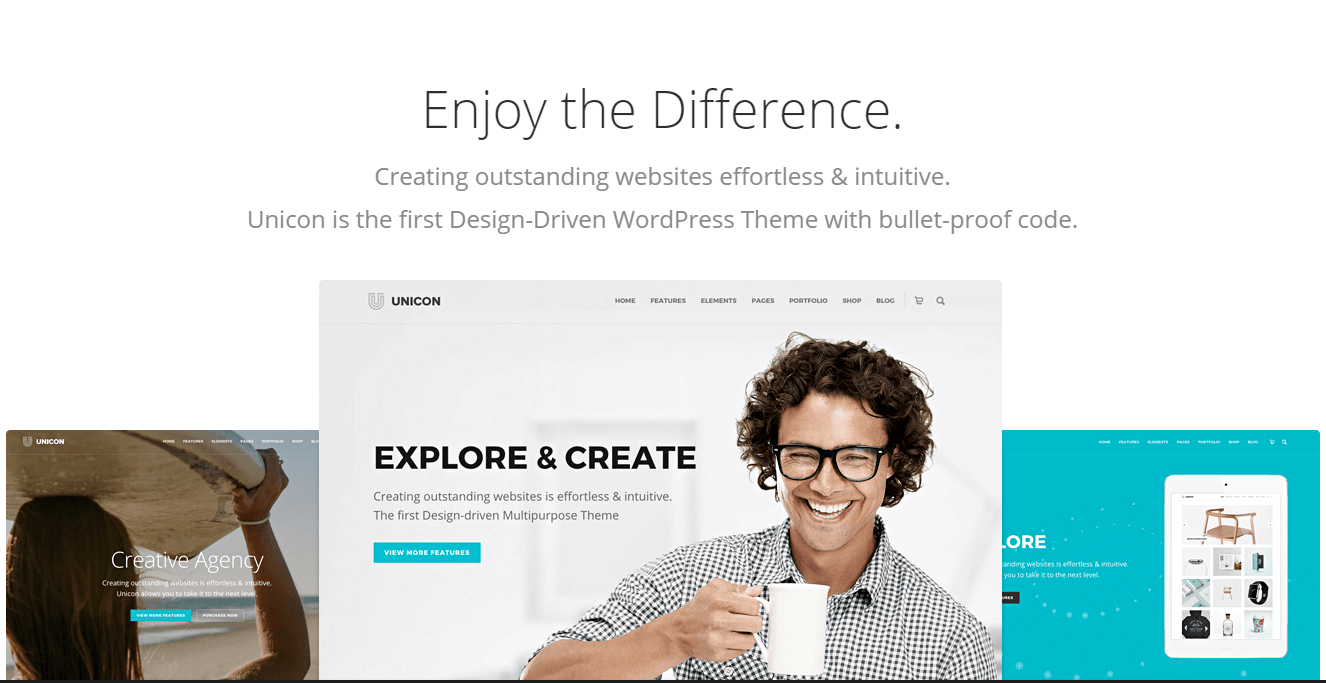Screenshot of a minimalistic promotional webpage for the Unicon WordPress theme. The page features a clean design with a white background and black text. At the top, bold text reads "Enjoy the Difference" and "Creating Outstanding Websites Effortlessly and Intuitively," followed by a statement: "Unicon is the first design-driven WordPress theme with bulletproof code." Below this text, there are three images aligned horizontally at the bottom of the page.

The central image is the largest and highlights the Unicon website's home page. It depicts a clean interface with the Unicon logo at the top left and navigation tabs including Home, Features, Elements, Pages, Portfolio, Shop, Blog, along with icons for a shopping cart and a search magnifying glass. The central image also features a section with the text "Explore and Create" alongside a smiling man with curly hair, glasses, and a mug. A blue button labeled "View More Features" is visible near the text.

To the left, a smaller image showcases a "Creative Agency" theme with a partial view of a woman holding a surfboard, seen from behind. The text accompanying this image is small and not entirely legible.

To the right, another smaller image with a blue-toned background displays various products available on the Unicon website, accompanied by some unreadable text.

Overall, the screenshot serves as an advertisement for the Unicon WordPress theme, emphasizing its user-friendly design and versatility.